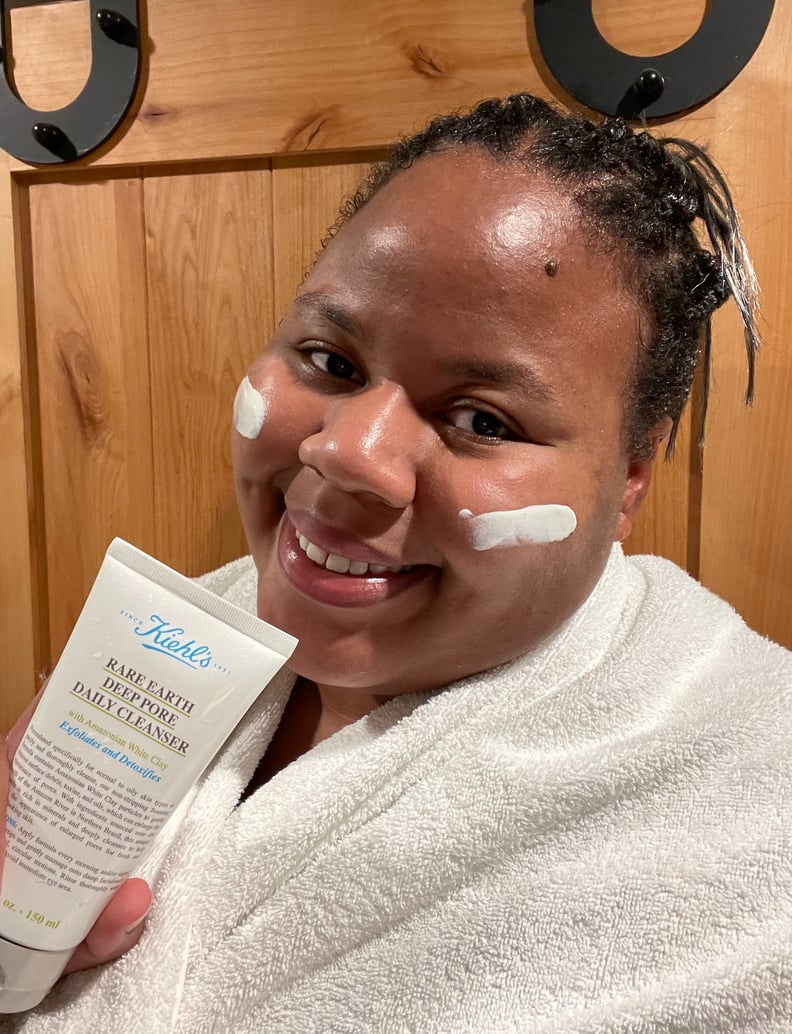The image features a young African-American woman standing in front of a rustic wooden door with two black circular hooks mounted on it. She is smiling broadly, her full cheeks accentuated by her rosy lips. Her hair is styled in cornrows, tied back tightly with a stray strand hanging down the right side of her face. She has a noticeable mole above her left eyebrow. The woman has applied two streaks of Kiehl's Rare Earth Deep Pore Daily Cleanser on her cheeks, the white contrasts vividly against her darker skin tone. She holds up a white tube of the same product in her right hand, showing the brand name "Kiehl's" in blue at the top and the product description "Rare Earth Deep Pore Daily Cleanser" in bold black text below. She is draped in a white towel that sits around her shoulders, and the image is cropped just above this. The brown wooden door behind her features vertical panels in the center flanked by horizontal grain panels on the top and sides. Her overall appearance suggests contentment and satisfaction with the skincare product she is promoting.